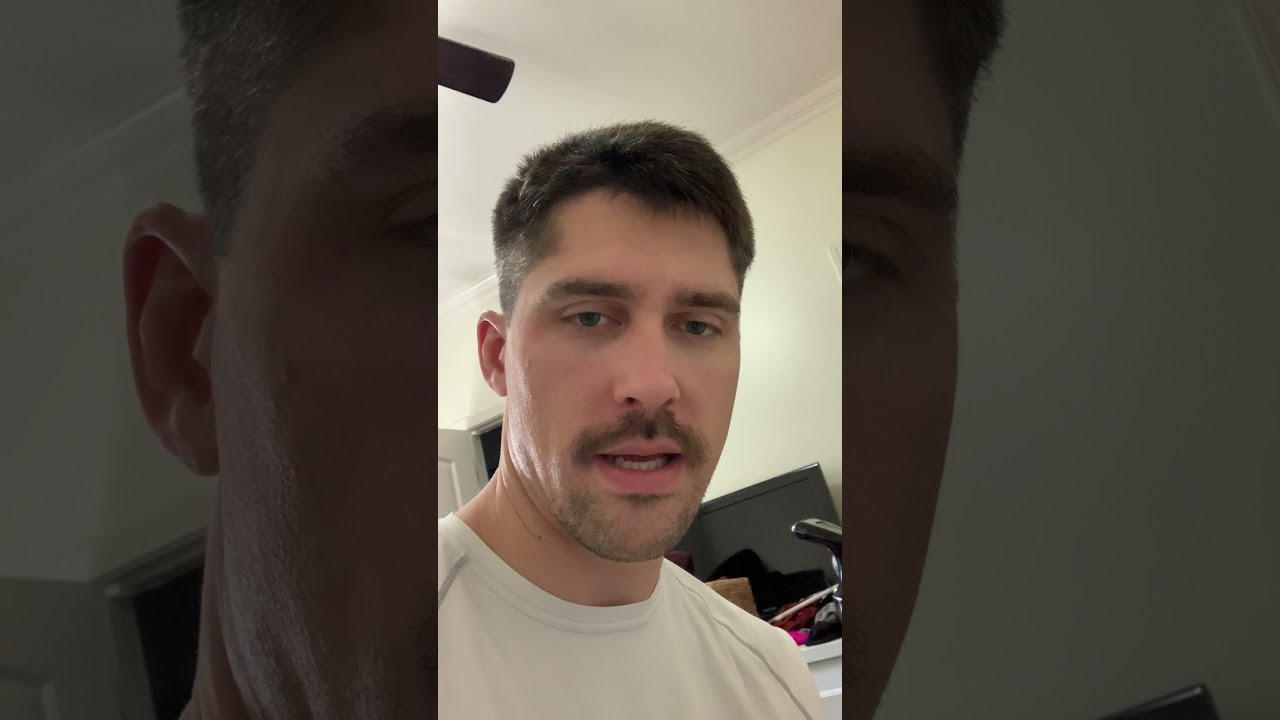This image captures a selfie of a young Caucasian man, possibly in his late 20s or early 30s, looking directly at the camera, perhaps recording a video or taking a photo. He has short, brown, spiky hair that's closely shaved on the sides and slightly longer on top. His facial features include thick brown eyebrows, gray eyes, a newly grown mustache, a light goatee, and a small soul patch under his lower lip. He sports a white, athletic tri-fit shirt. The setting appears to be a bedroom with white walls and a white ceiling adorned with crown molding. There is a flat-screen TV visible over his right shoulder, and part of a fan blade is seen in the upper left corner of the image. Scattered objects, including possibly an exercise bike, are in the background. The image composition features close-up, darkened and enlarged versions of the man's face flanking the central portrait on both the left and right sides, creating a triptych effect in a landscape orientation.